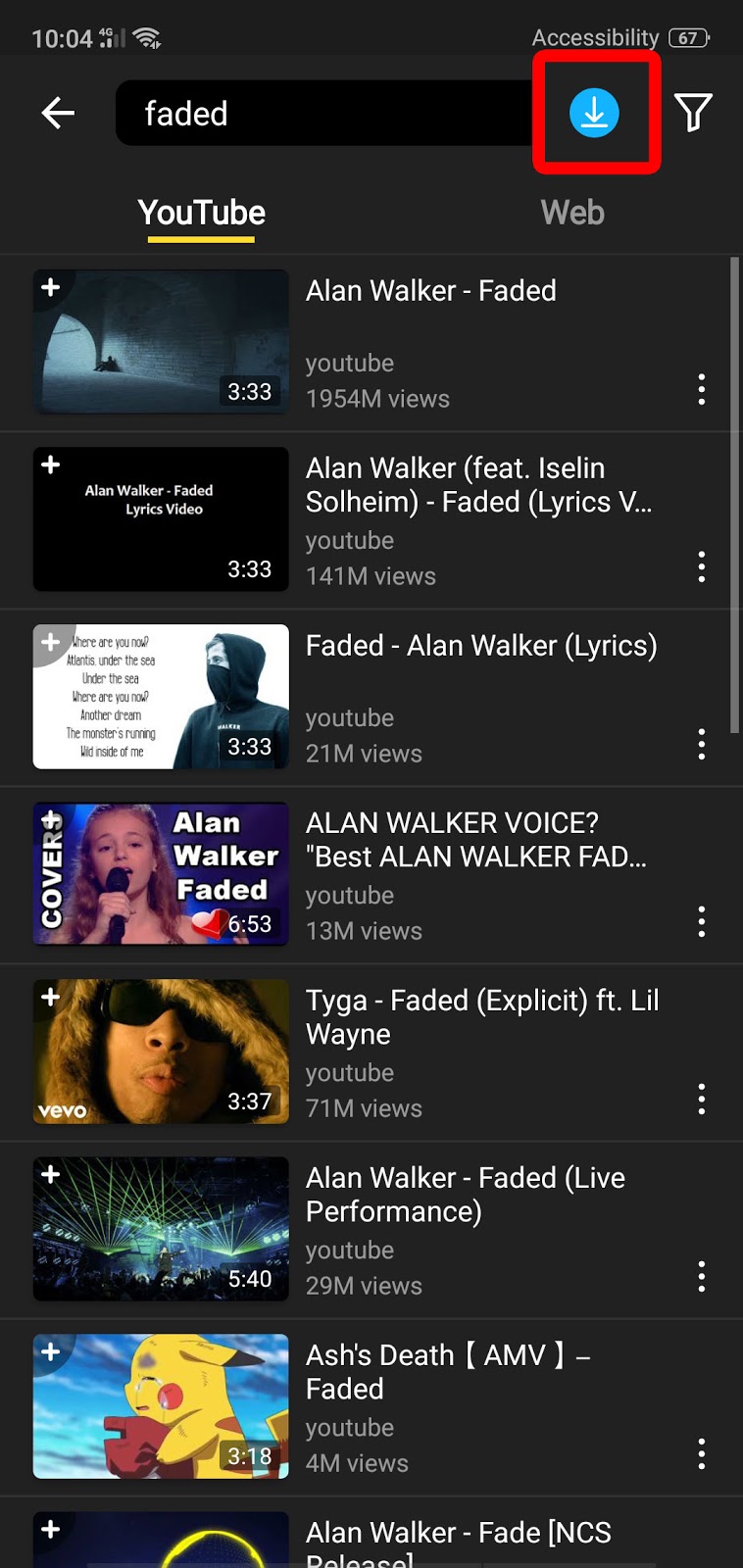**Caption:**

The image is a detailed screenshot from a mobile device, showcasing a YouTube search results page. At the top of the screen, the mobile UI displays several icons on a dark gray background. From left to right, these icons include the time (10:04), a signal strength indicator showing two out of four bars, a full Wi-Fi connectivity icon, the word "Accessibility" in text, and a horizontal battery icon indicating a 67% charge.

Beneath these icons, the navigation bar features from left to right: a left-pointing arrow, a black rectangular box with the word "faded" in white text, and a blue circle with a white download icon, which is highlighted with a red, rounded-corner square outline presumably added by the user for emphasis.

Below the navigation bar, two tabs labeled "YouTube" and "Web" are displayed, with "YouTube" currently selected as indicated by a yellow underline.

The main content comprises search results for the term "faded" on YouTube, arranged in rows. Each result includes a thumbnail on the left, textual information on the right, and a three-dot menu icon at the bottom right. The first result features a blue-toned image resembling tornadoes, with a duration of 3:33 and a plus icon in the top-left corner. The text to the right reads:

- **Title:** Alan Walker - Faded
- **Source:** YouTube
- **Views:** 1,954 million
- **Menu Icon:** Three-dot menu

The second result showcases a black thumbnail with "Alan Walker featuring Iselin Solheim - Faded (Lyrics) V..." in white text, 141 million views, and also includes the familiar three-dot menu icon.

Similar patterns follow for the remaining search results, all pertaining to the keyword "faded," each with distinctive thumbnails and varying views but maintaining the consistent layout.